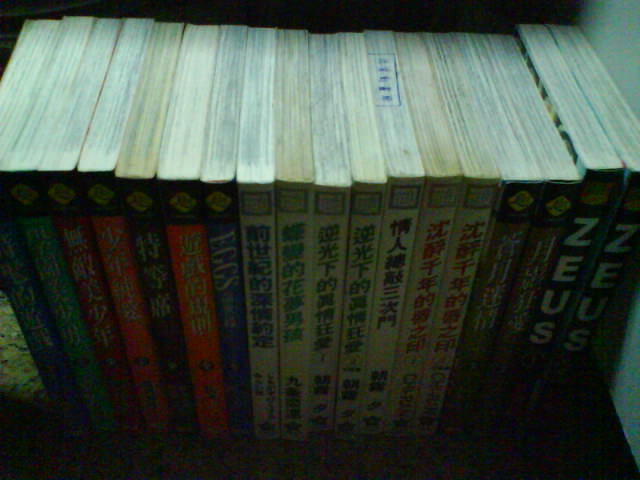The image depicts a dimly lit photograph of a row of around 20 books neatly lined up on a shelf. The image is grainy, likely taken in a very dark setting, which has introduced a high degree of noise obscuring finer details. The books are illuminated from above, making the tops of the pages more visible while the spines remain shadowed. The spines are adorned with titles almost exclusively in Asian characters—likely Chinese or Japanese—making them difficult to identify. However, a few spines bear English text: one says "ECCS," and two books at the far right prominently feature "ZEUS" in white letters. The books are predominantly of uniform thickness, and two distinct logos are visible on top of the bindings: a yellow circle and a square with a golden border and white center. The spines display a varied palette, transitioning from darker colors like blue, green, red, and orange on the left, through several white spines with colorful lettering in the middle, to dark, almost black spines on the right. The seven books on the left and the next seven seem to form two distinct series, possibly graphic or light novels, suggesting a grouping by publisher. One book near the middle has a blue ink stamp on the top of its pages, adding a unique detail to this collection.